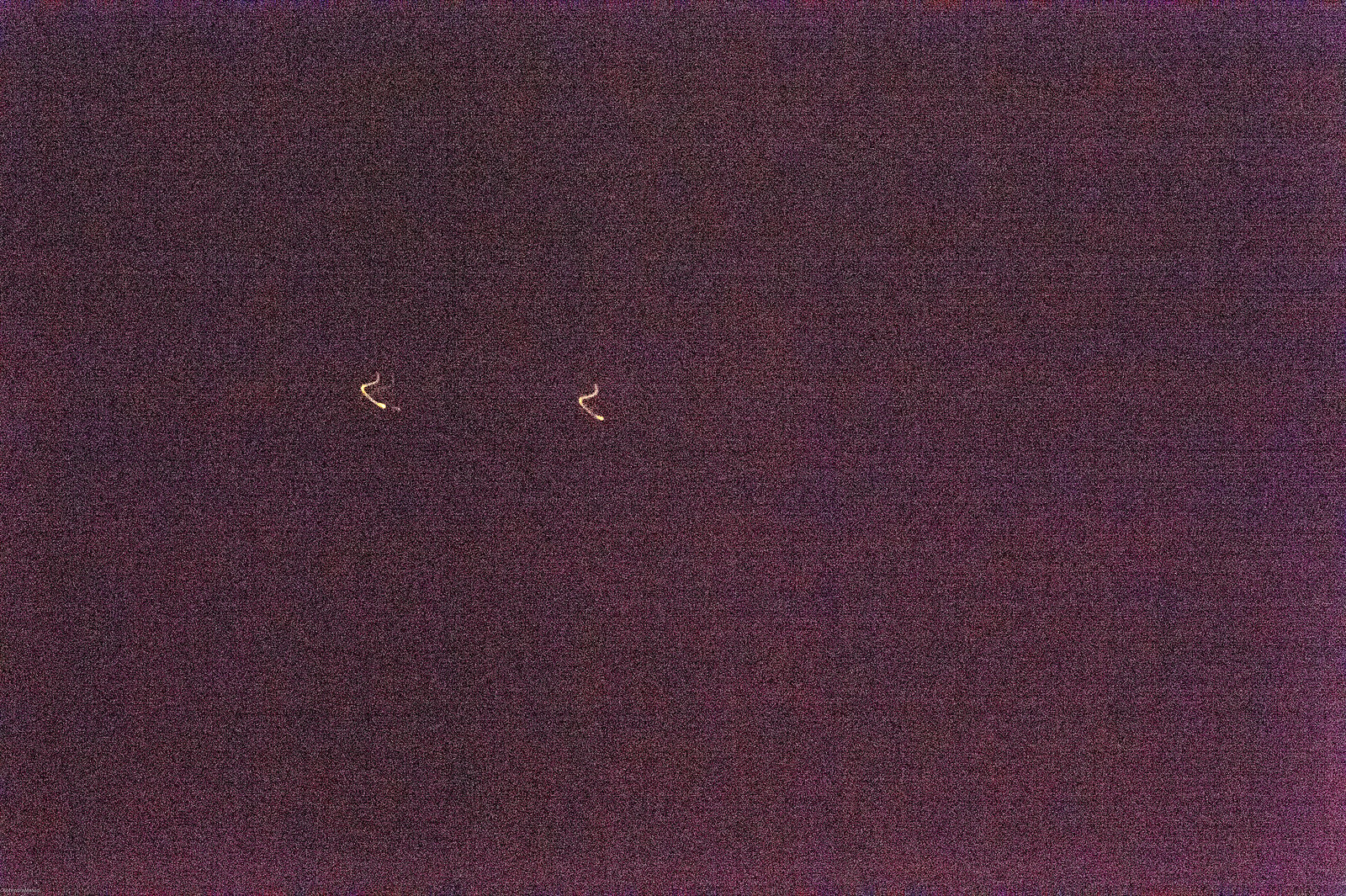This is a square photograph featuring a reddish-black material. The material appears darker at the top and lighter towards the bottom right corner, where there is a more pronounced reddish tinge. The image has a grainy texture and appears to be speckled, with white speckles scattered throughout. In the bottom right corner and extending across the bottom, the image is noticeably overexposed, resulting in a very bright, washed-out appearance. In the center of the material, there are two distinctive white shapes resembling halves of a triangle or upside-down V's, one located towards the left-middle and the other nearer the center. These shapes have straight edges along the top, with the left one appearing to have a sort of reflection. Additionally, there are two lines in the very center of the image, described as yellowish-golden and shaped like the letter C. Despite the overexposure and graininess, these elements provide a focal point within the photograph.